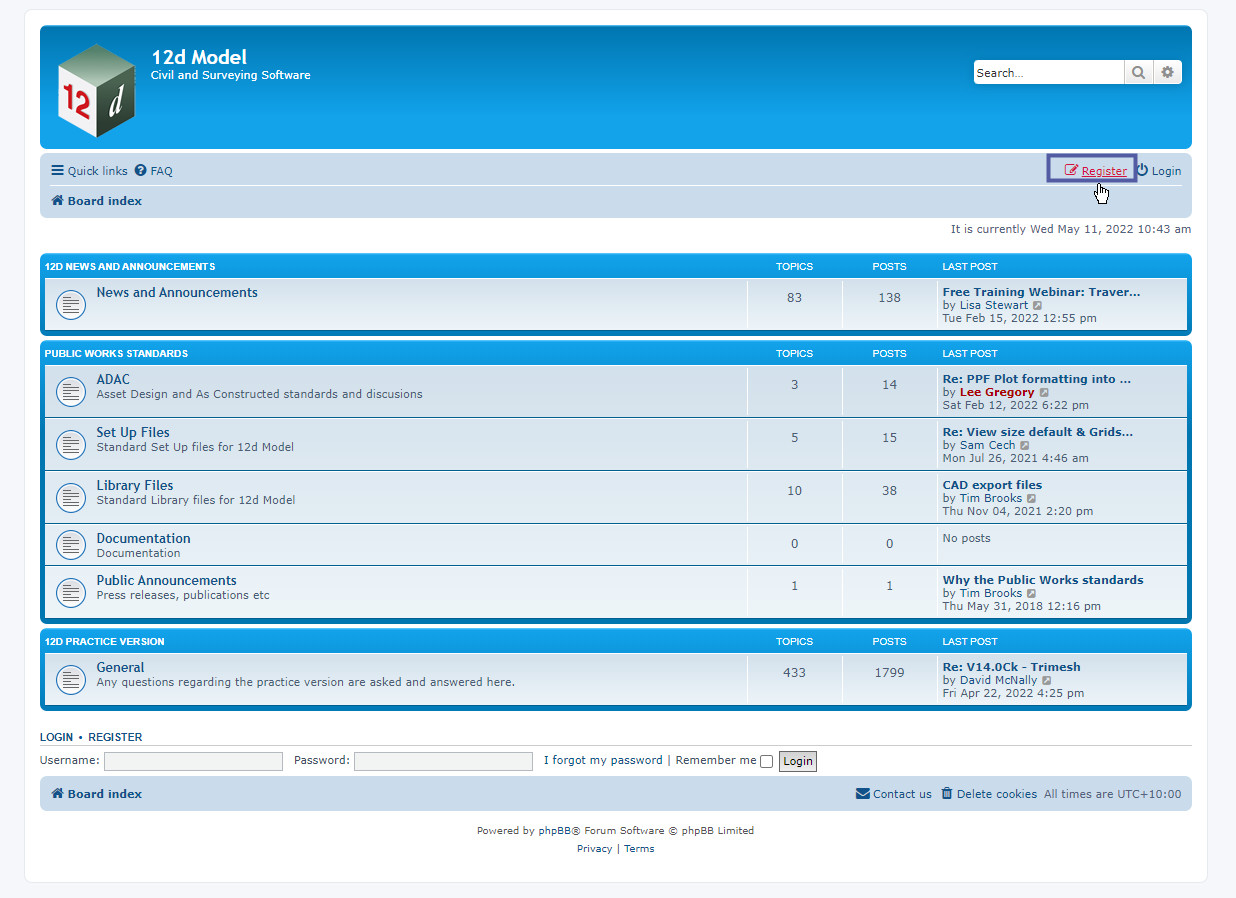Screenshot of a website displaying a "12D model" interface. At the top of the screen, there's a prominent title "12D model" alongside a visual representation of a cube labeled "12D." In the upper right corner, there's a clickable search bar, and just below it, a series of navigational options or action buttons. These include various sections such as news and announcements, setup files, each indicating the number of items available within. Further down, there's a form area where users can enter their username, password, and additional information to access the site.